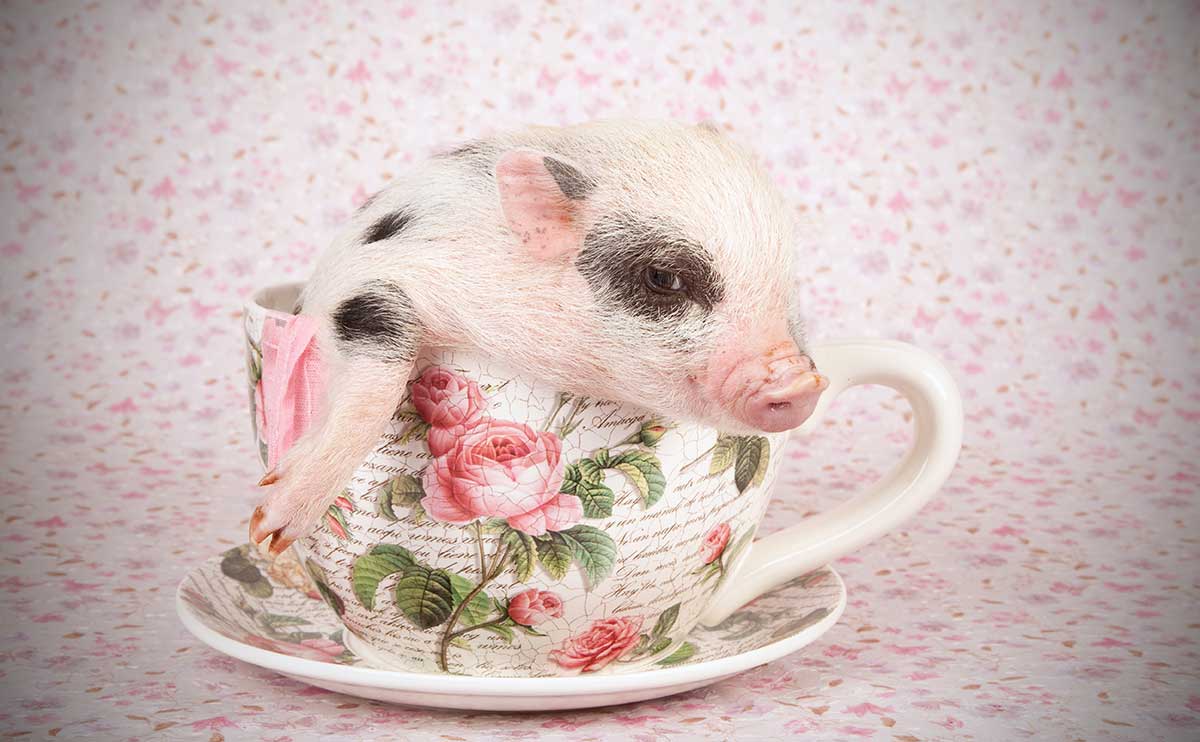The image is a beautifully artistic depiction of a baby piglet nestled in a vintage teacup that sits atop a matching saucer. The background is adorned with a soft, slightly blurred print of white coupled with delicate pink and mauve flowers, which imparts a whimsical, dream-like quality to the scene. The four corners of the image gradually transition to a dark grey, enhancing the central focus where the lighting is more pronounced.

The teacup and saucer feature elegant calligraphy in horizontal lines, complemented by a classic rose motif with rich pink petals and deep green leaves accented with lighter shades. The piglet, the heart of the artwork, is oriented to the right. Its adorable front right paw dangles over the edge of the teacup, giving it a curious and playful expression. The piglet's ear, nose, and feet exhibit a soft pink hue, while a distinctive patch of black fur adorns the area around its right eye and includes a charming tiny black spot within its ear. Flecks of black fur speckle its back, contrasting with the rest of its predominantly white coat, adding to the detailed and captivating nature of the image.